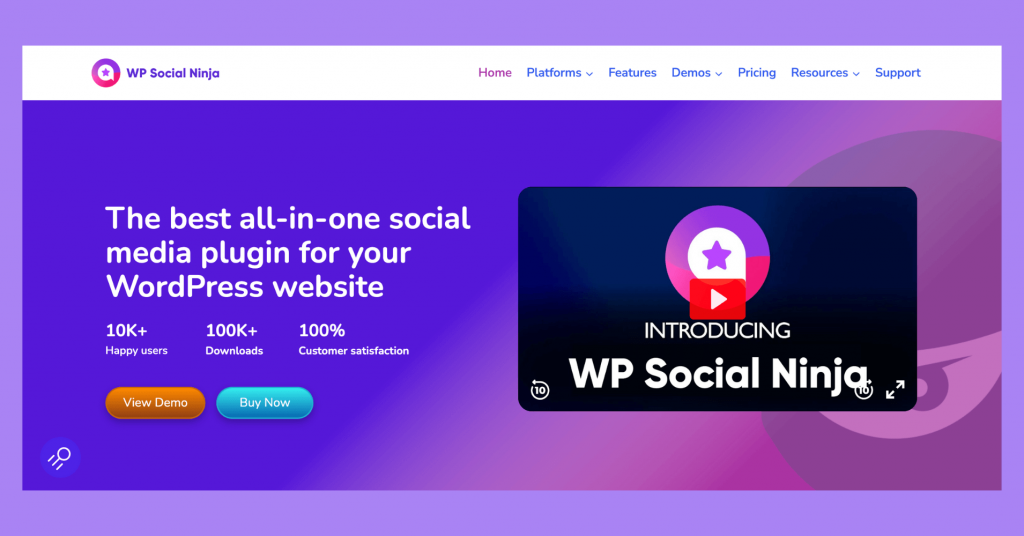The advertisement for WP Social Ninja features a stylish lavender border with the product name prominently displayed in purple. The navigation menu includes tabs labeled 'Home' in pink, 'Platforms' in blue, and 'Features,' 'Demos,' 'Pricing,' 'Resources,' and 'Support,' all in blue. The background transitions from white to a gradient of deep blue on the left, lightening to a pinkish hue on the right.

At the forefront of the design, white text announces it as "the best all-in-one social media plug-in for your WordPress website," boasting "10K+ happy users," "100K+ downloads," and "100% customer satisfaction." Below this, a series of call-to-action buttons include an orange "View Demo" and an aqua "Buy Now." Adjacent to these is a black box labeled "Introducing WP Social Ninja," which seems to contain a video, indicated by a play button overlaying their vibrant logo. The logo itself transitions from pink to lavender and finally to purple.